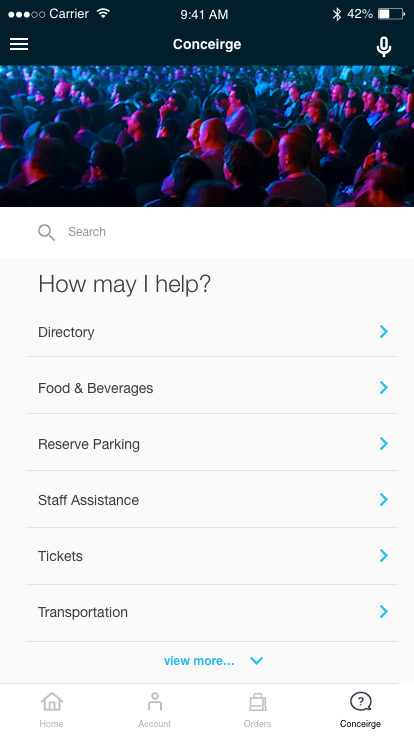This image is a screenshot from a cell phone. The top header bar is dark navy blue, with white text and icons, including the battery percentage on the top right, Bluetooth symbol, and signal strength on the top left. The word "carrier" is next to the signal strength icon, and the time is centered in the middle. Beneath the time, in large, bold white font, it says "Concierge." On the leftmost edge of this header bar, there is a three-bar hamburger menu icon, and on the rightmost edge, there is a white microphone symbol.

Below the header, the main content of the screenshot is a picture taken from behind a crowd at a concert, with the crowd illuminated by dark blue and purple lights, showing the backs of people's heads.

Beneath the concert image, there is a list with expandable sections, titled "How may I help?" This list includes different categories separated by thin horizontal gray lines. Each section has a blue caret on the right edge, indicating that it can be expanded. The categories listed are "Directory," "Food and Beverage," "Reserve Parking," "Staff Assistance," "Tickets," and "Transportation." At the bottom center of the list is the blue text "View more."